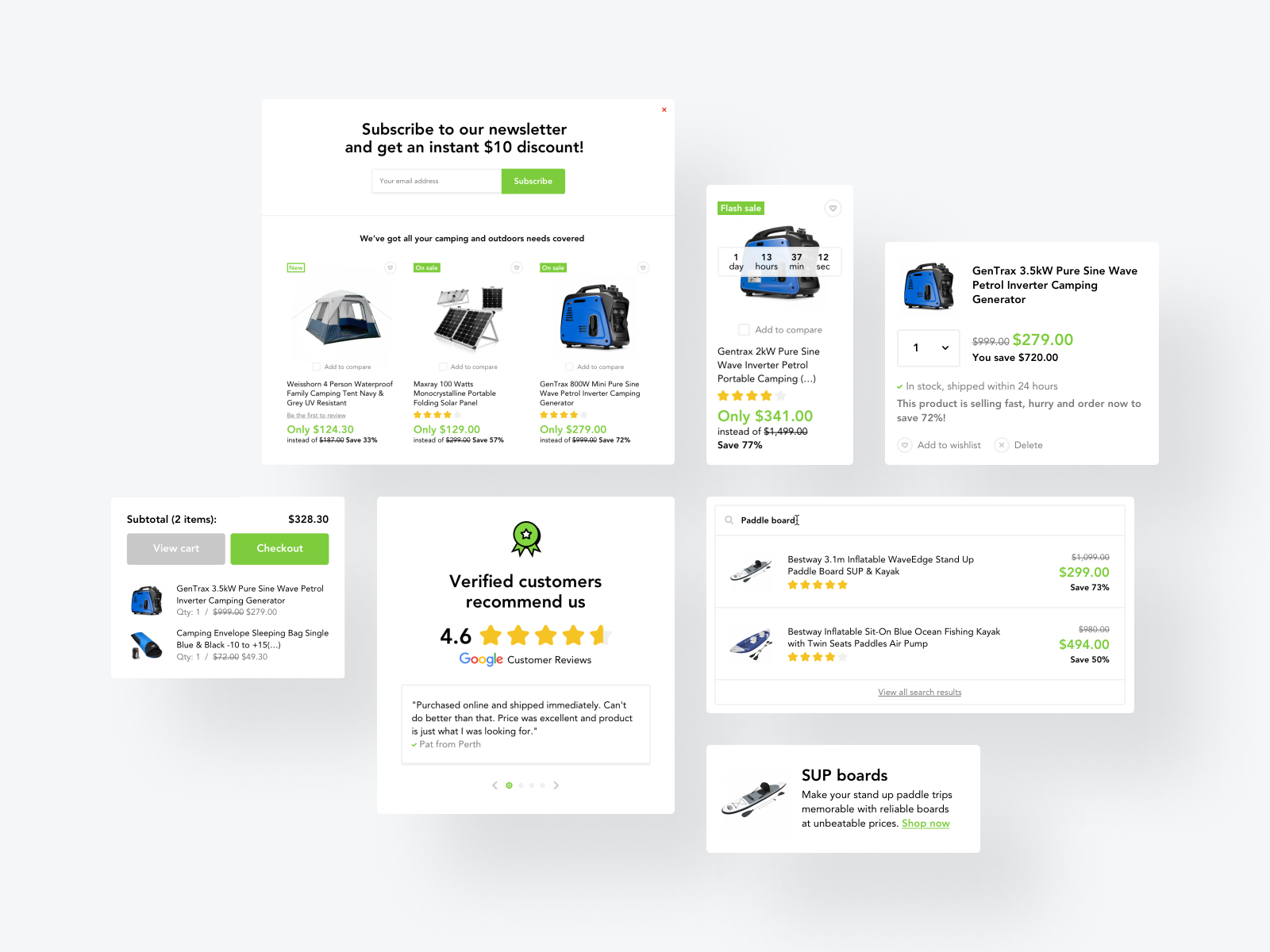The image showcases an assortment of various promotional white boxes, each featuring different products and offers. The most prominent box, positioned centrally, invites viewers to "subscribe to our newsletter" with the incentive of an instant $10 discount. This message is presented in large, bold text and includes a red 'X' in the top-right corner, allowing users to close the prompt. Below the text field for entering an email address and a "subscribe" button, there's a display of three camping-related products.

The first product is highlighted with a green "new" tag in the top left corner. It features an image of a navy and gray two-tone camping tent with visible windows. The caption beneath it reads, "Westhorn four-person waterproof family camping tent in navy gray," priced at $124.30, which is a 33% discount from its original price of $187.00.

Next is the "Max Ray 100 watts monocrystalline portable folding solar panel," priced at $129.00, discounted from $299.00. This product has a rating of four stars.

The third featured item is a camping generator priced at $279.00. Adjacent to it, a flash sale is ongoing for a "Generax" generator, marked down to $341.00 from $1500.00, with a countdown timer showing the time remaining for the deal. Another generator, a 3.5 kilowatt model, is listed for $279.00 in a box to the right.

Additionally, there is a section dedicated to paddle boards, promoting "SUP boards" aimed at enhancing stand-up paddle trips with reliable and competitively priced boards. A box on the left highlights a verified customer review from Google, with a testimonial beneath it. Another smaller box to the left lists items a customer intends to purchase: a Generax 3.5 kilowatt generator and a camping envelope sleeping bag, totaling $328.30.